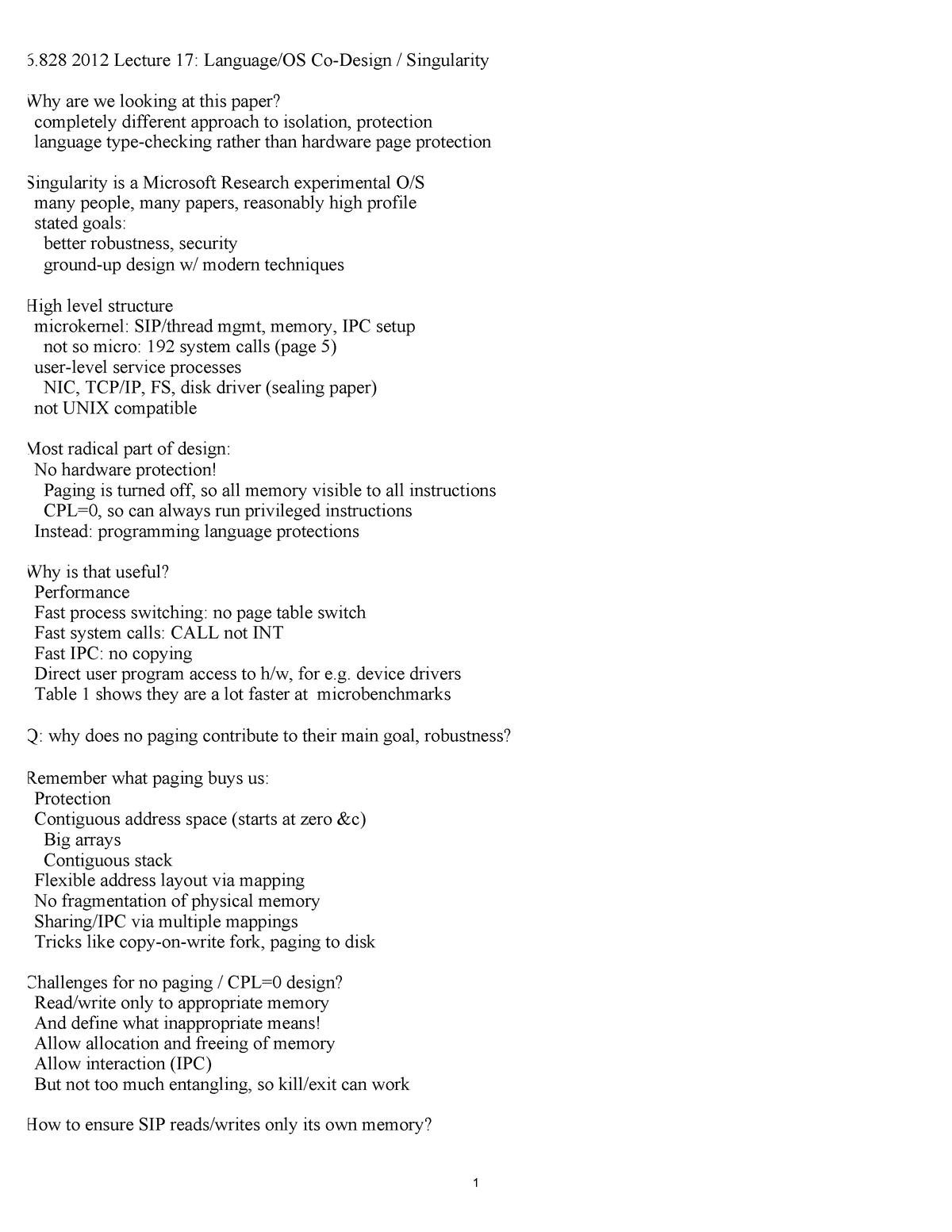**Detailed Caption:**

This screenshot captures the contents of a detailed lecture slide from the year 2012, specifically Lecture 17, centered on the topic of language-based operating system (OS) co-design with a focus on Singularity, an experimental OS developed by Microsoft Research.

At the top left of the slide, key information is displayed:
- Numeric identifier: "5,828"
- Lecture reference: "2012 Lecture 17"
- Topics: "Language OS Co-design / Singularity"

The main content of the slide addresses the innovative approach Singularity takes towards OS design, summarizing its key aspects:
- Purpose: To evaluate a completely different approach to system isolation and protection, emphasizing language type checking over traditional hardware page protection.
- Context: Singularity is a significant research project with multiple contributors and extensive publication, aiming to enhance robustness and security through modern design techniques.

The high-level structure of Singularity is outlined as:
- Core: Microkernel coupled with simple thread management (SLP/thread MGMT), memory and Inter-Process Communication (IPC) setup.
- Notable Detail: Despite being labeled micro, the kernel contains 192 system calls.
- System Services: User-level service processes handle network interface controllers (NICs), TCP/IP, file systems (FS), and disk drivers, as referenced in the sealing paper.

A standout feature of Singularity is its departure from traditional hardware protection:
- Radically, paging is disabled, exposing all memory to all instructions, where all software runs at the highest privilege level (CPL=0).
- This leverages programming language protection rather than hardware mechanisms, offering significant performance advantages:
    - Fast process switching and system calls by avoiding page table switching and incremental operations.
    - Fast IPC without data copying.
    - Direct hardware access for user programs, exemplified by device drivers.

The performance benefits are quantitatively illustrated in Table 1, which shows Singularity outperforming traditional systems in various micro benchmarks. 

This slide provides a comprehensive overview of Singularity's design philosophy and its potential performance benefits, positioning it as an innovative rethinking of OS architecture.